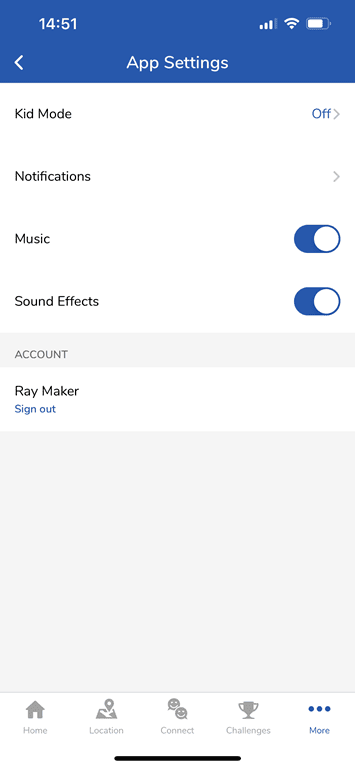A detailed screenshot of a mobile device's settings menu is displayed. The screen is predominantly three tones: dark blue, white, and black, with an additional light gray box at the bottom.

At the top of the screen is a dark blue status bar, which shows the time as 14:51, signal strength at 3 out of 4 bars, Wi-Fi strength at 4 bars, and the battery level at approximately 75%. Below this status bar is a left arrow icon followed by the title "App Settings."

The central part of the screen is a white box with black text. The menu items listed in this box are "Kid Mode" (with "Off" in blue letters to its right), "Notifications" (with a right-facing gray arrow to its right), "Music," and "Sound Effects." Both "Music" and "Sound Effects" have a blue oval switch with a white circle indicating they are turned on.

Below this menu section is a gray bar labeled "Account," followed by a white bar with black text "Raymaker," and below it, blue text reading "Sign out."

The bottom portion of the screen is a light gray box, which takes up most of the remaining screen space. Within this box is a white navigation bar with gray icons labeled "Home," "Location," "Connect," "Challenges," and a blue "More" icon represented by three horizontal dots. At the very bottom, there is a slider bar.

The interface is user-friendly, combining clear visual elements with functional settings options.